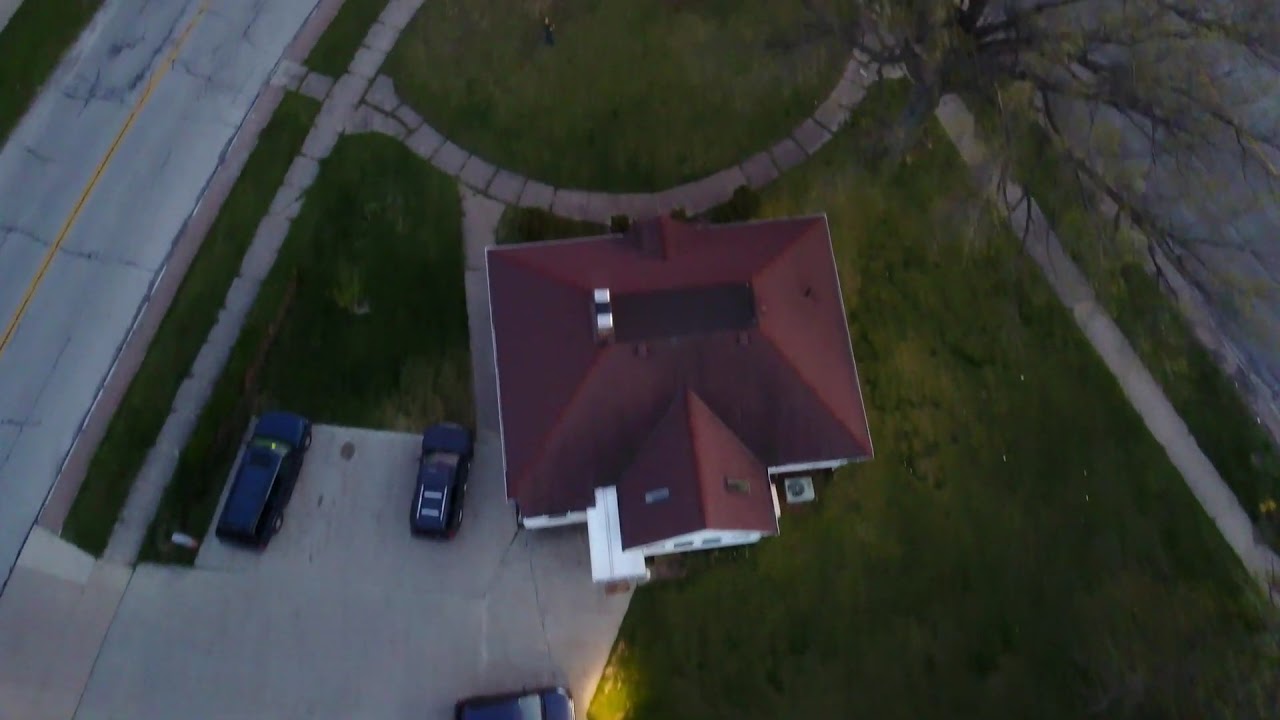The aerial image, likely taken from a drone, showcases a well-maintained residential property with distinctive features. Central to the image is a two-story house with a prominent red roof and white walls, possibly accented with brick at the base. The roof includes a smaller triangular section at the front, hinting at the house's multi-story nature. Surrounding the house is a network of stone walkways forming an interesting curved shape, particularly notable in the front and along each side. A large green yard, featuring a well-tended lawn and sparse shrubbery, frames the house. A sizeable and mostly barren tree, potentially signaling early spring or fall, stands near the back alongside a semicircular stone pathway. The left side of the image reveals a substantial parking area made of stone pavement, accommodating three blue SUV-type vehicles, highlighting the expansive nature of the driveway. Bordering the property to the left is a two-lane road with a yellow center line, providing clear access to the residence.